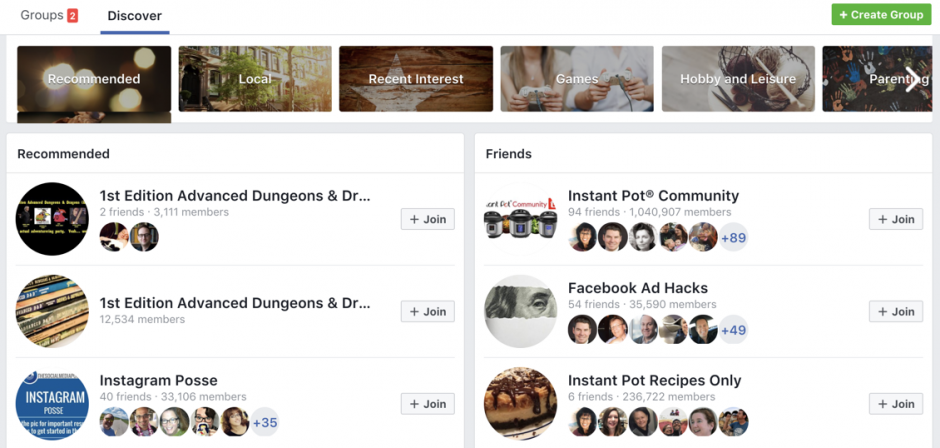This screenshot captures the Discover section of Friends and Groups on Facebook. In the top left corner, there are two tabs: 'Groups' with a red notification icon displaying the number 2, and 'Discover,' which is currently selected and underlined in blue. In the top right corner, there's a green rectangle with white text that reads 'Create Group.'

Below these tabs, a series of images with overlaid white text represents different categories. These categories include 'Recommended' on a sparkly background, 'Local' on a picture of a building, 'Recent Interest' with a star on a wooden background, 'Games' featuring two people playing video games, 'Hobby and Leisure' with an array of sports balls, and 'Parenting,' which shows colorful handprints on a wall.

Further down, there are two main sections. The left section is titled 'Recommended' and lists three group suggestions: '1st Edition, Advanced, Dungeons, and Drrrrrrrrrrr,' '1st Edition, Advanced, Dungeons, and Drrrrrrrrrrrrrrrrrrrrrrrrrrrrrrrrrrrrrrrrrrrrrrrrrrrrrrrzzzzzzzzzzzz,' and 'Instagram Posse.' On the right, under the 'Friends' header, it lists 'Instapot Community,' 'Facebook Adhax,' and 'Instapot Recipes Only.'